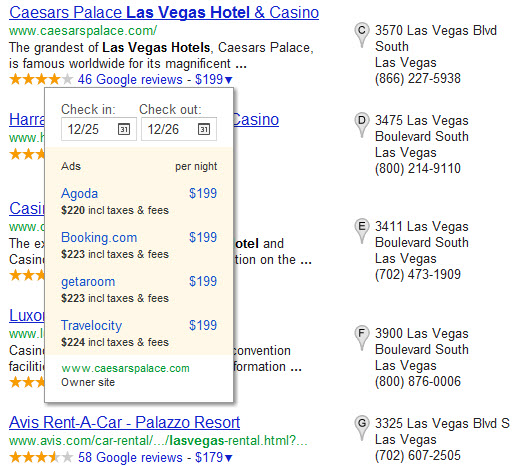The image depicts a search results page for accommodations in Las Vegas. 

On the right side, a column lists various addresses and phone numbers for different locations. On the left side, the page showcases five search results, some of which are partially covered by a rectangular box displaying check-in and check-out dates. The search results are as follows:

1. The first visible result is for "Caesars Palace Las Vegas Hotel and Casino." The description reads, "The grandest of Las Vegas hotels, Caesars Palace, is famous worldwide for its magnificent..." This listing features a four-star review and a price of $199.
  
2. Beneath it, there are three more search results that are mostly obscured by the rectangular box.

3. The final visible search result is for "Avis Rent-A-Car at Palazzo Resort." This listing includes an Avis address, star rating, and a price of $179, along with a pull-down arrow for more details.

The rectangular box covering some of the search results displays the following information: "Check-in: 12/25, Check-out: 12/26," and mentions pricing sources such as Agoda, Working.com, Get A Room, and Travelocity.

On the far right, the column details the addresses and phone numbers of five different places in Las Vegas.